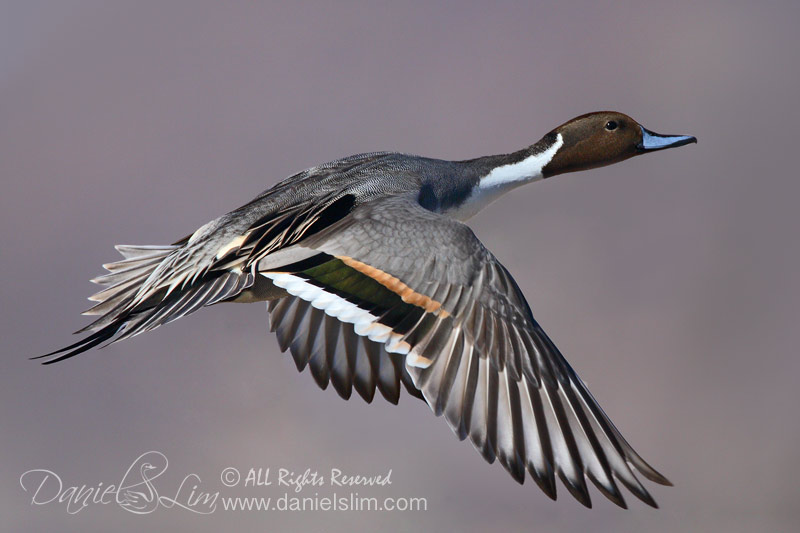The image features a highly realistic representation of a bird, possibly a goose or duck, mid-flight against a purplish-grey or mauve background that resembles a business card or promotional graphic. The bird's distinctive coloration includes a blue beak, a dark brown or black head with a black eye, and a white stripe running down the front of its neck. Its body and wings exhibit a mix of black, white, grey, and brown feathers, with the wings spread wide. The bird is positioned in profile, with its head angled towards the upper right corner of the image.

In the bottom left corner, in white or light grey lettering, is the artist's signature "Daniel Slim," written in cursive, with a unique logo incorporating a small drawing of a duck or bird within the letters "L" and "S." Below the signature is a copyright notice stating "All rights reserved" and the website "www.danielslim.com." The overall image is crisp, detailed, and appears almost like a photograph despite potentially being a painted or drawn artwork.